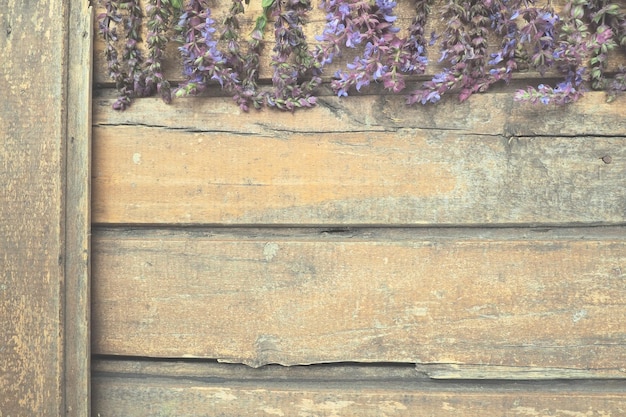This image captures a beautifully weathered, aged wooden structure, possibly a fence, barn stall, or the side of a building. The horizontal wooden planks, in varying hues of gray, tan, cream, orange, and brown, are cracked and distressed, showcasing rich color variations and a rugged texture. These horizontal boards, four in total, are supported by a vertical piece of wood on the left side of the photo, which is notably less cracked but uniformly aged, with visible nail heads securing the structure. Near the top of the image, delicate purple flowers, which appear to be lavender, with green stems cascade over the planks, accentuating the rustic charm of the scene. There is no signage or text, ensuring the focus remains on the natural beauty and intricate details of the weathered wood and flowering plants. The photo exudes a sense of timelessness and serenity, perfectly capturing the quiet elegance of decay and nature's gentle reclamation.